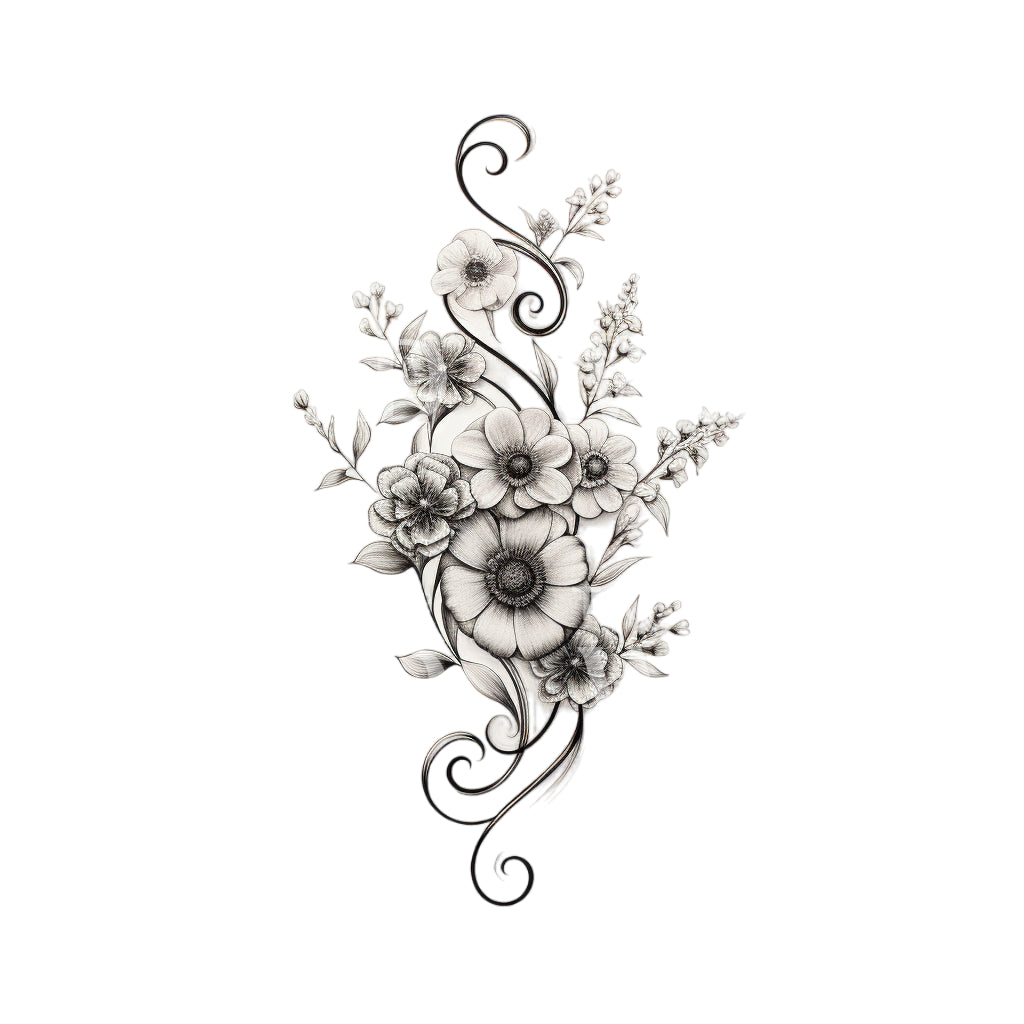This is a detailed, black-and-white illustration or possibly a fine line drawing of a stylized floral arrangement set against a plain white background. The centerpiece features a large daisy-like flower with a dark, seed-filled center. Surrounding it are six smaller flowers, adding up to a total of seven flowers, arranged primarily in a vertical manner. Above the central cluster, two additional flowers extend upward, with one slightly to the left and another on top. Intricate, swirling lines and curves intertwine gracefully with the flowers, adding a whimsical touch to the design. These curves also extend downward and laterally across the composition. Leaves and twigs with budding blossoms protrude from the sides, enhancing the intricate detailing. The overall artwork has an Art Nouveau and Victorian flair, making it suitable for a decorative piece, possibly a tattoo design, wallpaper, or even a coloring book. The meticulous and artistic rendering showcases impressive drawing skills, capturing a sense of delicate beauty.